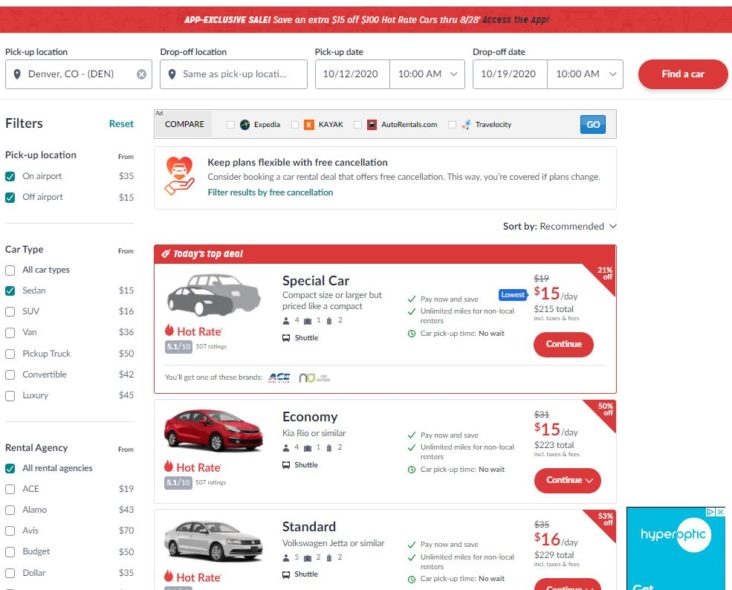This image showcases a detailed view of a car rental website interface. 

At the very top, a prominent red banner spans the width of the screen, advertising an "App Exclusive Sale" in bold white text. The promotion offers an additional $15 off rentals over $100 for "Hot Red Cars" through August 28th, accessible via the app, indicated in black text.

Beneath the banner, the site provides input fields for rental specifics. The pick-up location is set to Denver, with the drop-off location defaulted to the same. The pick-up date is specified as October 12th, 2020, at 10 AM, with the drop-off scheduled for October 19th, 2020, at 10 AM. A conspicuous red button labeled "Find a Car" in white text is positioned to the right.

Below these fields, filter options are laid out, showing that both "On-Airport" and "Off-Airport" pick-up locations are selectable, priced at $35 and $15 respectively. The chosen car type filter is set to "Sedan" at $15. The rental agency filter is inclusive of all agencies.

An advertisement strip underneath emphasizes flexibility, promoting free cancellations with a reminder that booking such deals is beneficial if plans change. 

The "Hot Rate" section highlights today’s top deal, featuring a "Special Car" of compact size or larger, priced like a compact at $15 per day. Additional options include an economy car, such as the Kia Rio or a similar model, priced at $15 per day, and a standard car like the Volkswagen Jetta or a similar model, priced at $16 per day.